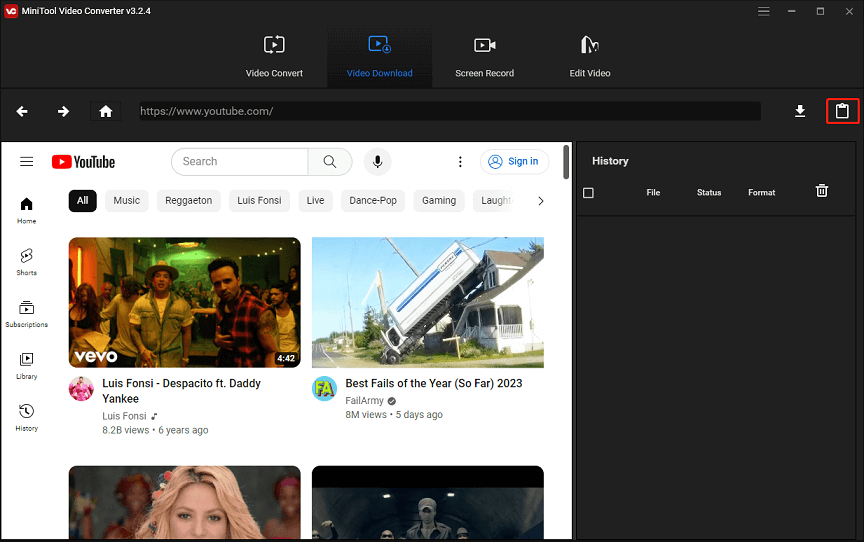This screenshot showcases a YouTube page with a predominantly black background. In the top left corner, a logo featuring the letter "V" in white against a red background is partially visible, which likely pertains to a software named "miniTool Video Converter." Beneath the logo, the text "Video Convert" appears, with "Convert" highlighted in blue, though it's difficult to read due to its size. Next to it are the options "Screen Record" and "Edit Video."

Further down the left side, white left and right arrows, along with a home button, are visible. The search bar displays the URL "https://www.youtube.com," and at the far right of this bar, there are save and rectangular icons, with the latter being outlined in red.

Below the toolbar, the YouTube interface is visible, complete with the YouTube logo and standard navigation icons. Four video thumbnails are displayed prominently:
1. **Top Left:** "Despacito"
2. **Top Right:** "Best Fails of the Year So Far 2023"
3. **Bottom Left:** Shakira's "World Cup South Africa" music video
4. **Bottom Right:** The partially visible top half of a black and white icon.

These elements together make for a detailed and informative snapshot of the YouTube browsing experience amidst the context of using a video conversion software.